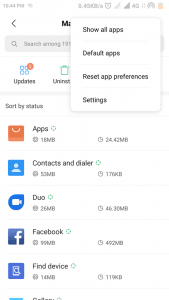The image showcases a smartphone settings screen with a predominantly white background. 

- **Top Section:**
    - The current time is displayed on the top left, reading "10:44 PM". 
    - There is series of icons indicating network and device status:
        - An alarm clock symbol.
        - Two bars symbols, possibly indicating signal strength.
        - A "4G" symbol.
        - The battery icon is halfway filled, suggesting a 50% charge.
    - There is also a data indication of "0.45 kilobytes per W".

- **Overlay Section:**
    - The screen has an overlay featuring black text options such as:
        - "Show all apps"
        - "Default apps"
        - "Reset app preferences"
    - A title/header labeled "Settings" appears at the top left, accompanied by a back arrow.
    - There is a section labeled "MA" in bold black text, partially obscured by the overlay.
    - A search bar partially reads "social number 191".
    
- **Notification and Icons Section:**
    - A red notification badge with the number "5" appears next to an update icon on the left.
    - An "Uninstall" option partially visible below the update icon.
    - Text indicating "Store by status" in dark gray.
    - A list of app icons arranged vertically includes:
        - Apps (default)
        - Contact and dialer
        - Duo
        - Facebook
        - Find device
    - The right side of the list shows the size of each app in gray text and their respective storage usage:
        - 18 megabytes
        - 53 megabytes
        - 26 megabytes
        - 900 megabytes
        - 14 megabytes